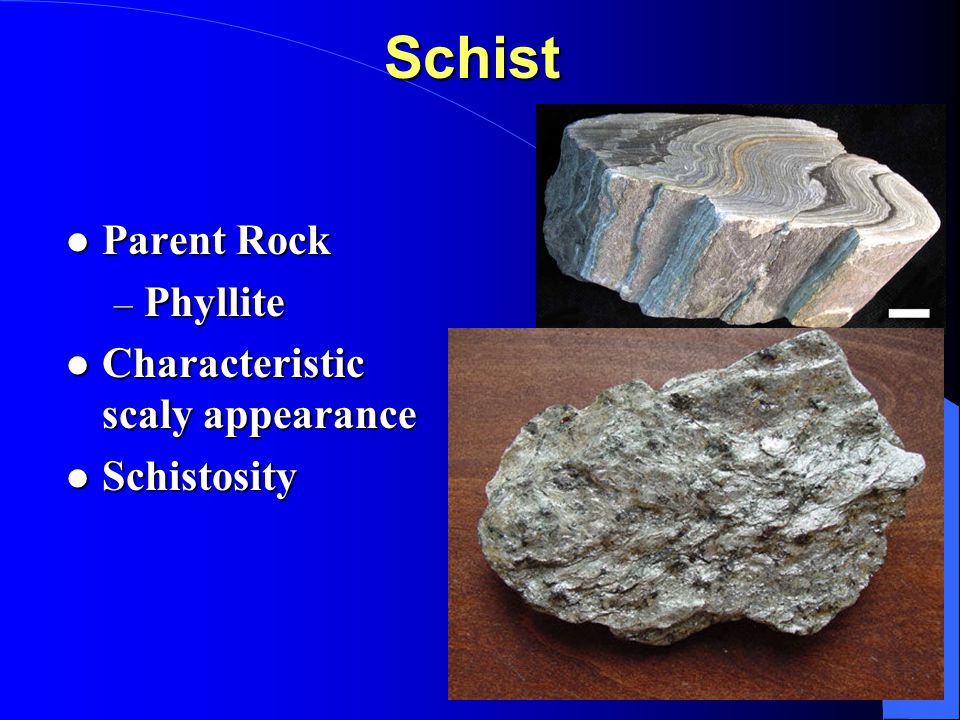The PowerPoint slide presents detailed information about the rock Schist against a blue gradient background, transitioning from a bright blue on the left to a darker blue on the right. The title "Schist" is prominently displayed at the top in yellow text. On the right side of the slide, two images of Schist are shown, stacked vertically. The upper image, set against a black background, features a cutaway cross-section of the rock, revealing its smooth, wavy internal structure. The lower image shows a more natural, complete piece of Schist placed on a wooden table, characterized by its gray color with black spots and jagged edges. The left side of the slide contains three white bullet points providing key information: the parent rock is Phyllite, the rock's characteristic scaly appearance, and the feature known as Schistosity.